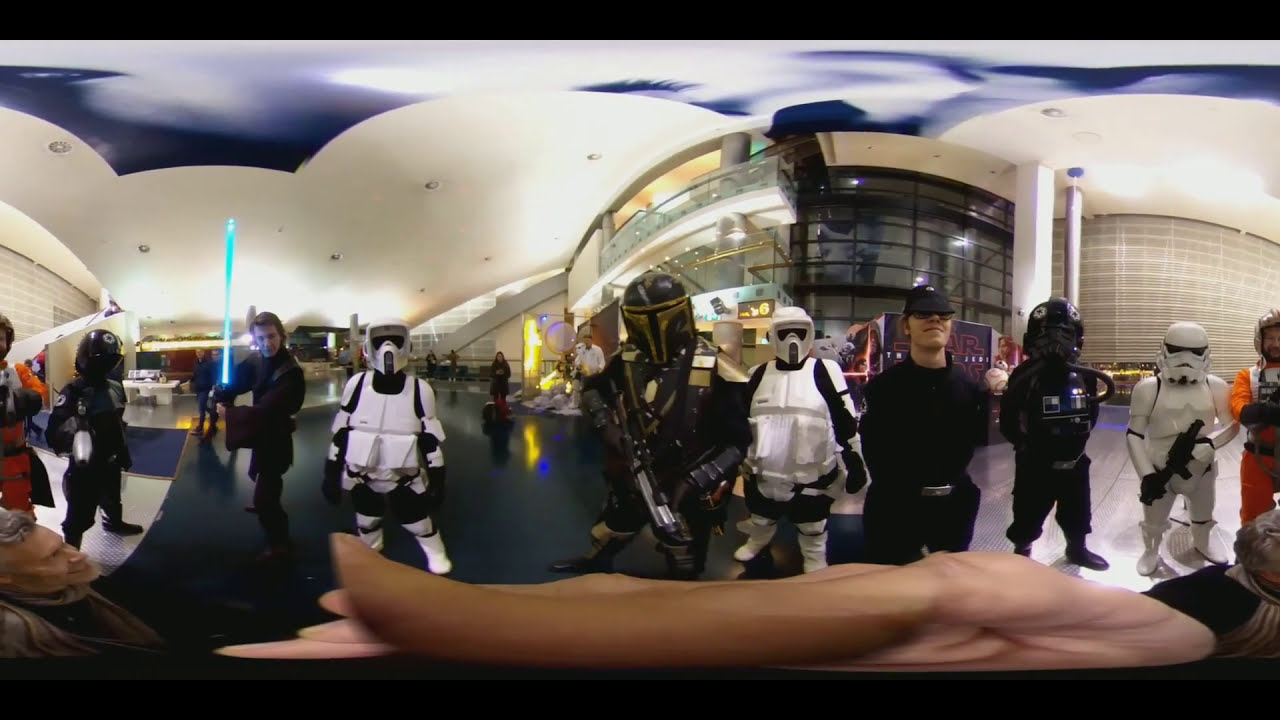The image is a horizontally aligned rectangular picture with black borders along the top and bottom edges. It appears to have been taken at a large-scale convention, possibly a Star Wars-themed event, held in a spacious venue with a high ceiling and prominent windowed walls. The setting includes an upstairs area accessible by stairs or an escalator, suggesting a multi-floor layout.

The background features various signs and posters, including prominently visible "Star Wars" branding. The foreground showcases a group of approximately ten individuals dressed in Star Wars costumes. On the far left stands a figure in black armor with a black helmet. Next to them is a person in all-black attire, holding a blue lightsaber, resembling Anakin Skywalker. Following them is a Stormtrooper. At the center of the image is another participant in black and gold armor flanked by another Stormtrooper.

Continuing to the right, there is another individual clad in black with a black visor, beside another figure in black armor. On the far right, a Stormtrooper holds a black prop gun, next to what appears to be a Star Wars fighter pilot in an orange jumpsuit. The floor tiles are predominantly black, contrasted by white walls and ceilings dotted with spotlights.

In the lower section of the image, there is a distorted and elongated view of someone's hand, likely a result of the wide-angle or 360-degree VR capture method used for the photo.